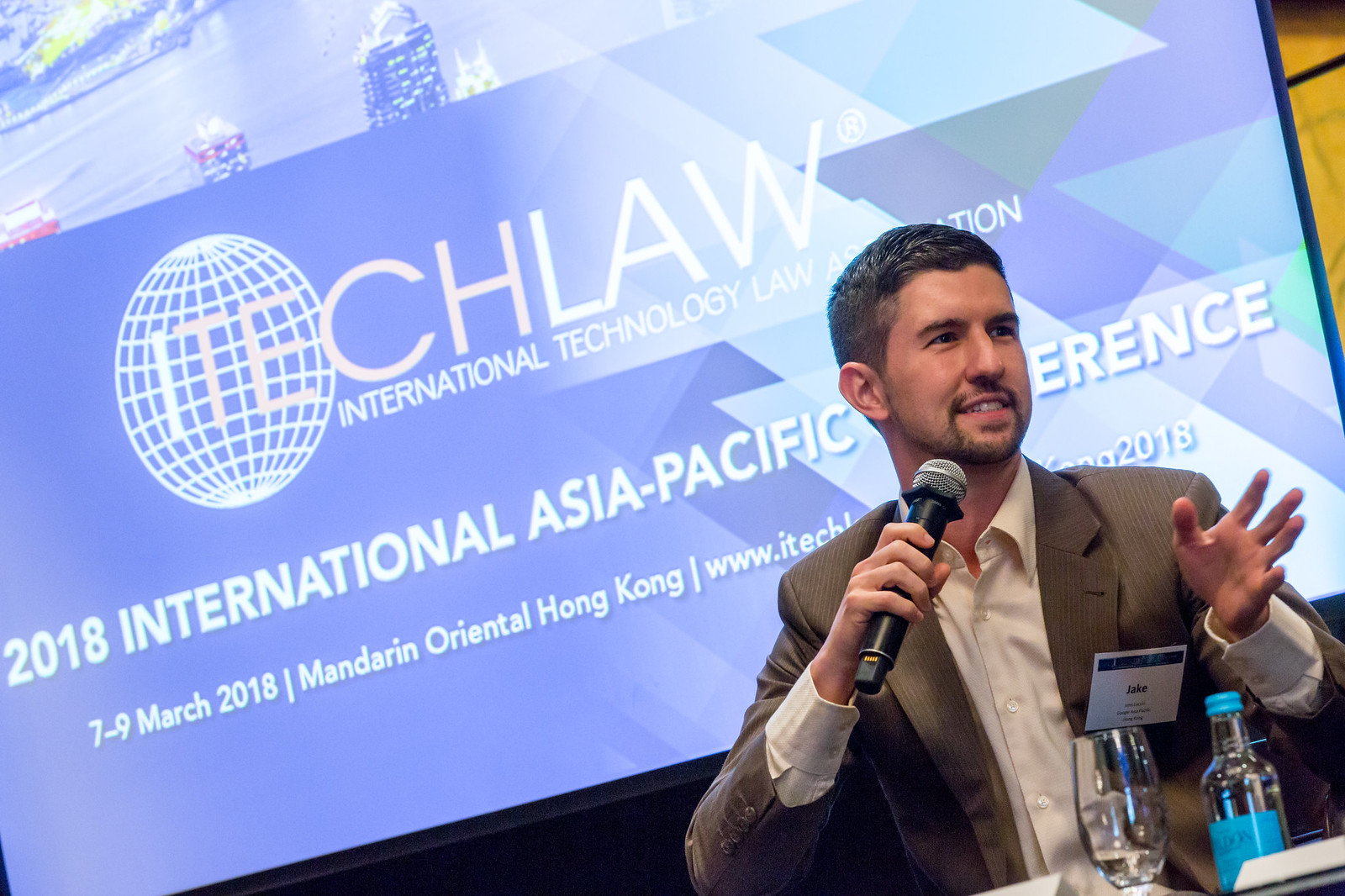In this detailed photograph, a young man is speaking at the 2018 International Asia Pacific Conference organized by the International Technology Law Association, held from March 7th to 9th at the Mandarin Oriental in Hong Kong. The man, seated in the lower right corner of the image, is a white male with neatly combed brown hair and a short brown beard resembling a goatee. He is dressed in a grayish-brown sport jacket over a white dress shirt and is wearing a name tag that reads "Jake." Jake is holding a wireless microphone in his right hand and gesturing with his left. In front of him, there is a nearly empty wine glass and a bottle of sparkling water with a blue label.

The conference details are displayed in the background on a large presentation screen, predominantly blue-colored with various textual elements. At the top of the screen is a stylized skyline, likely of Hong Kong, depicted against a body of water. A stylized grid-like globe with the letters "ITE" prominently displayed inside it appears just below. The text on the screen reads: "I Tech Law, International Technology Law Association," though some words are partially obscured by Jake's head. Further down, the screen mentions the event title and dates: "2018 International Asia Pacific Conference, 7-9 March 2018, Mandarin Oriental Hong Kong." The URL for the association is visible but partially blocked, displaying as www.itech... The image captures a dynamic moment as Jake engages with the audience, contributing to the lively atmosphere of the conference.